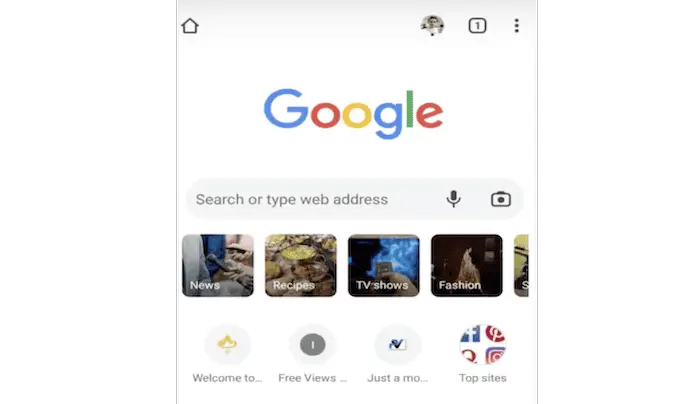This photo captures the Google homepage. The background is predominantly white. In the upper left-hand corner, there is a silhouette of a house icon. Moving to the upper right-hand corner, there is a round profile icon, rendered in black and white. Next to it, there is a square icon with a number one inside, followed by three vertically aligned dots.

In the center of the image, towards the top, the Google logo is prominently displayed in a larger font. Beneath the logo, there is a light gray search bar with the prompt, “Search or type a web address,” in gray text. Adjacent to the search bar, on the right, are a microphone icon and an image icon, indicative of voice search and image search functionalities respectively.

Directly below the search bar, spanning the middle section of the image, are several categorized squares labeled: News, Recipes, TV Shows, and Fashion. These squares likely represent popular search categories or shortcuts.

Towards the bottom, the text reads, “Welcome to Free Views,” followed by "just a moment and top stories," suggesting an introductory feature or news headline display.